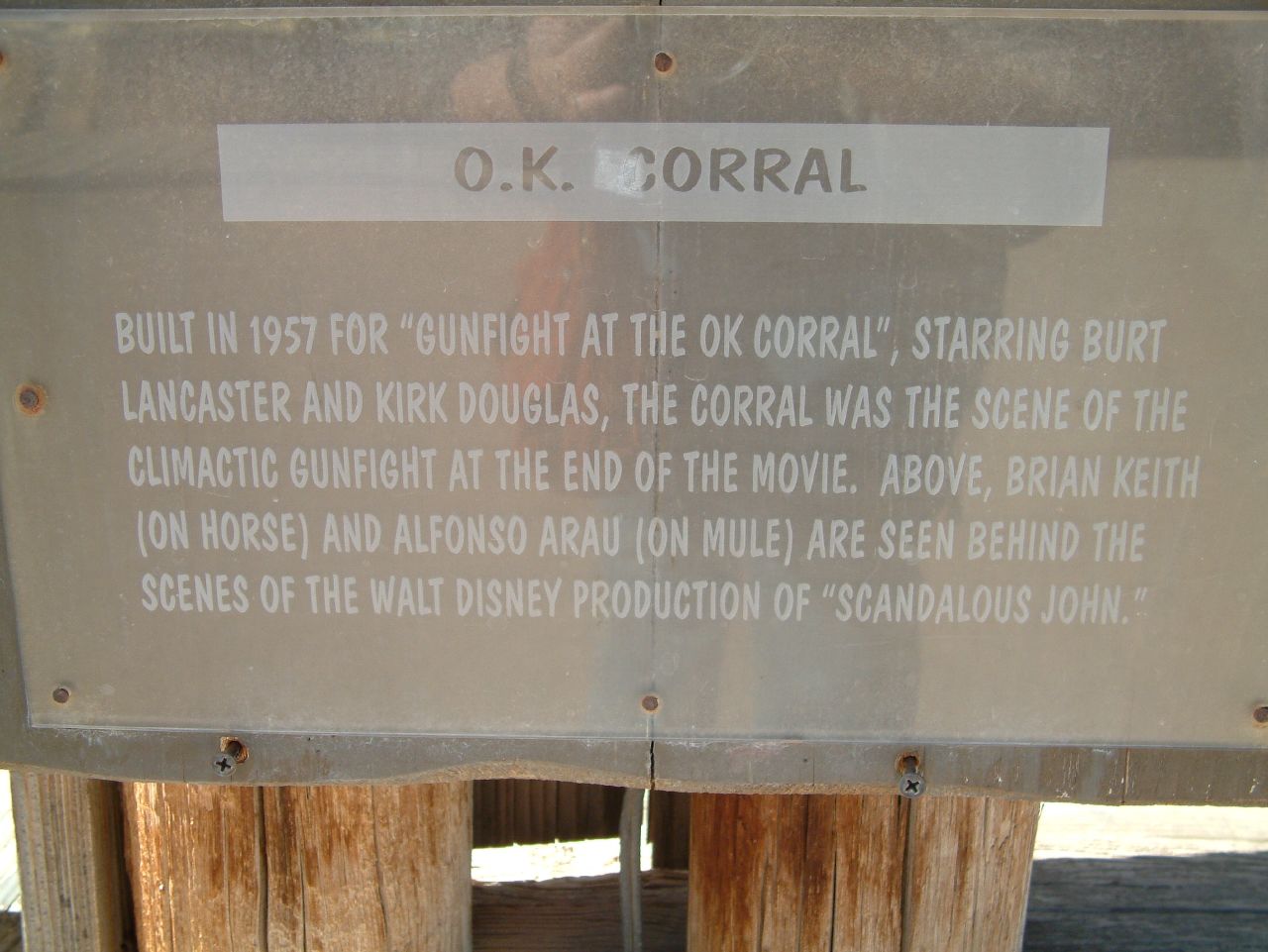The image captures an outdoor photograph of a vintage sign attached to two thick, weathered wooden columns with visible vertical cracks. These columns are set against what appears to be a wooden base in front of a fence, with light peeking through from the outside. The sign itself is a worn, cracked plastic plaque secured by rusty nails. At the very top of the sign, within a small white rectangle, the text "O.K. CORRAL" is displayed in grayish letters. Beneath this, in all-capitals white text, there is a detailed paragraph: "BUILT IN 1957 FOR 'GUNFIGHT AT THE O.K. CORRAL,' STARRING BURT LANCASTER AND KIRK DOUGLAS. THE CORRAL WAS THE SCENE OF THE CLIMACTIC GUNFIGHT AT THE END OF THE MOVIE. ABOVE, BRIAN KEITH (ON HORSE) AND ALFONSO ARRAU (ON MULE) ARE SEEN BEHIND THE SCENES OF THE WALT DISNEY PRODUCTION OF 'SCANDALOUS JOHN.'" The reflection of the photographer can be faintly seen in the plexiglass covering the sign, indicating they are carrying a red purse and wearing jeans.